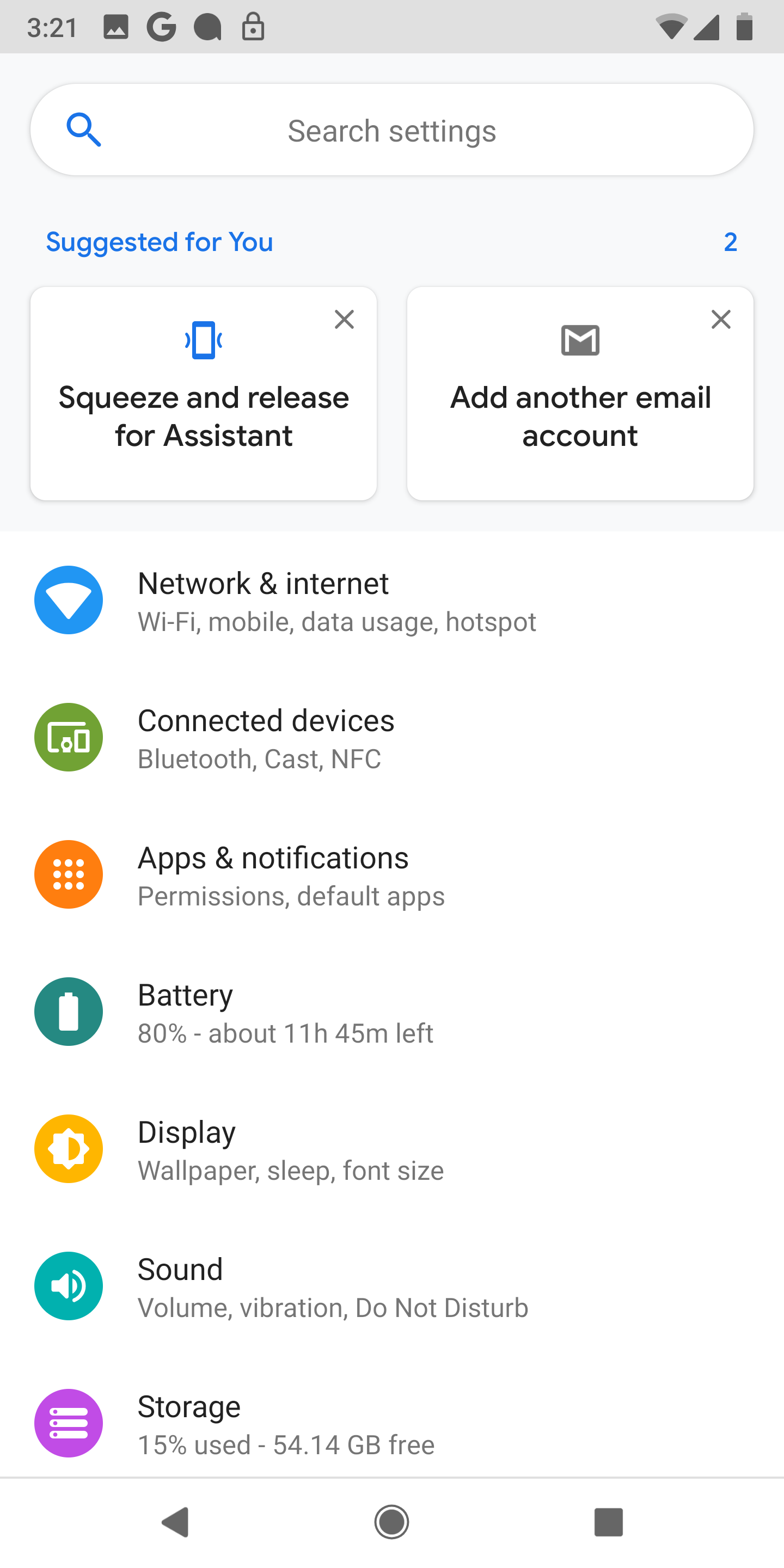A vertically rectangular screenshot of a cell phone display featuring the settings menu. The top banner, which is light gray with dark gray prints and icons, shows the current time as 3:21. Just below this, there is a slightly horizontally rectangular very light gray box with a "Search settings" bubble prominently displayed. Underneath, in blue text, it reads "Suggested for you," followed by two side-by-side boxes labeled "Squeeze and release for assistance" and "Add another email account." The main background of the screenshot is white, displaying various icons and selections typically found in a settings menu, such as "Network & Internet," "Connected Devices," "Apps & Notifications," "Battery," "Display," "Sound," and "Storage." At the bottom of the screen, three navigation icons are visible.